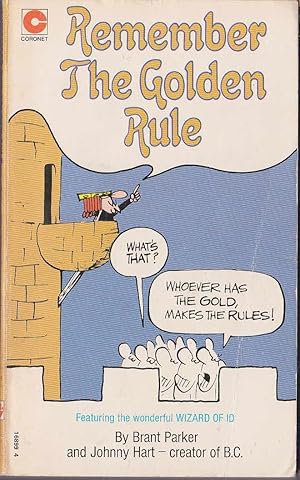The cover of the book features a cartoon illustration reminiscent of vintage newspaper comics. At the center of the image is a person resembling a king, identifiable by his red hair and small golden crown, standing on a balcony of a two-toned brick tower—brown on top and whitish at the bottom. The tower has a red "C" logo in the top left corner. The king, depicted in color, points upward as he speaks to a group of black-and-white line-drawn subjects gathered below. His speech bubble, written in golden text, reads "Remember the golden rule." The subjects respond with their own speech bubbles, asking "What's that?" and reacting with "Whoever has the gold makes the rules." At the bottom of the image, in blue text, it states "Featuring the wonderful Wizard of Id by Brant Parker and Johnny Hart, creator of B.C."